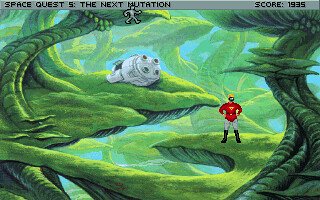Caption: 

A vibrant scene reminiscent of classic retro video games depicts a miniature, adventuring character navigating through a lush mushroom environment. Dominated by various shades of green, the landscape is adorned with mushrooms sprouting from ledges and rock formations richly carpeted in moss. The main character, dressed in a form-fitting red long-sleeved unitard, gray tights, and black boots, adds a striking contrast to the verdant backdrop. A distinctive yellow helmet obscures the character’s face, which appears to be darkened beneath the helmet's shadow. The background reveals a cylindrical, can-shaped spaceship with an open door, hinting at a crash landing. The bright blue sky overhead further emphasizes the surreal and adventurous atmosphere of this alien mushroom world.